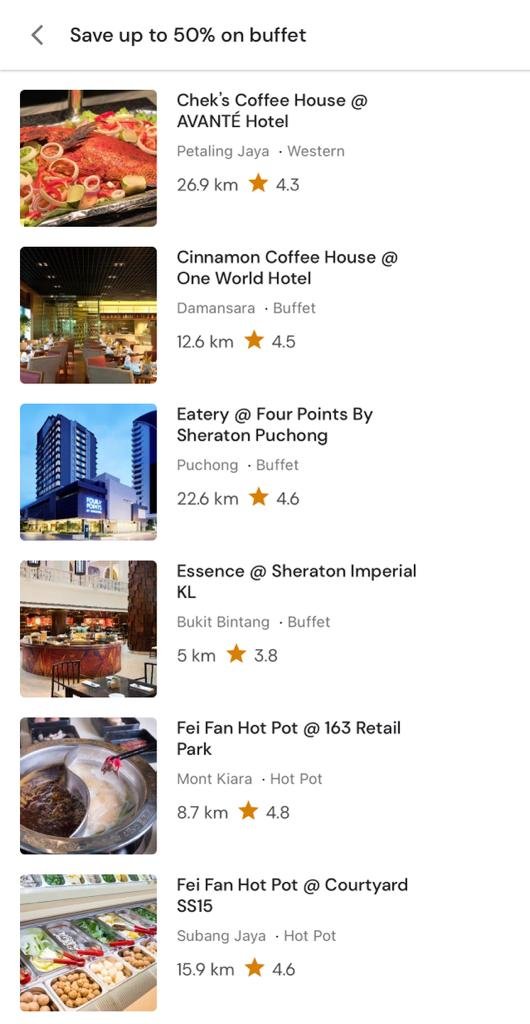The advertisement features an arrow pointing left with the message, "Save up to 50% on buffet," separated by a gray line. Below are images and descriptions of various dining options:

1. **Checks Coffeehouse at Avanti Hotel**:
   - Distance: 26.9 KM
   - Rating: 4.3 (Gold Star)

2. **Cinnamon Coffeehouse at One World Hotel**:
   - Distance: 12.6 KM
   - Rating: 4.5 (Gold Star)

3. **Eatery at Four Points by Sheraton Puchong**:
   - Distance: 22.6 KM
   - Rating: 4.6 (Gold Star)

4. **Essence at Sheraton Imperial KL**:
   - Distance: 5 KM
   - Rating: 3.8 (Gold Star)

5. **Fee Fen Hotspot at 163 Retail Park**:
   - Distance: 8.7 KM
   - Rating: 4.8 (Gold Star)

6. **Fee Fen Hotspot at Courtyard SS15**:
   - Distance: 15.9 KM
   - Rating: 4.6 (Gold Star)

The advertisement includes detailed rating information and distances for each establishment, along with their associated logos and images.